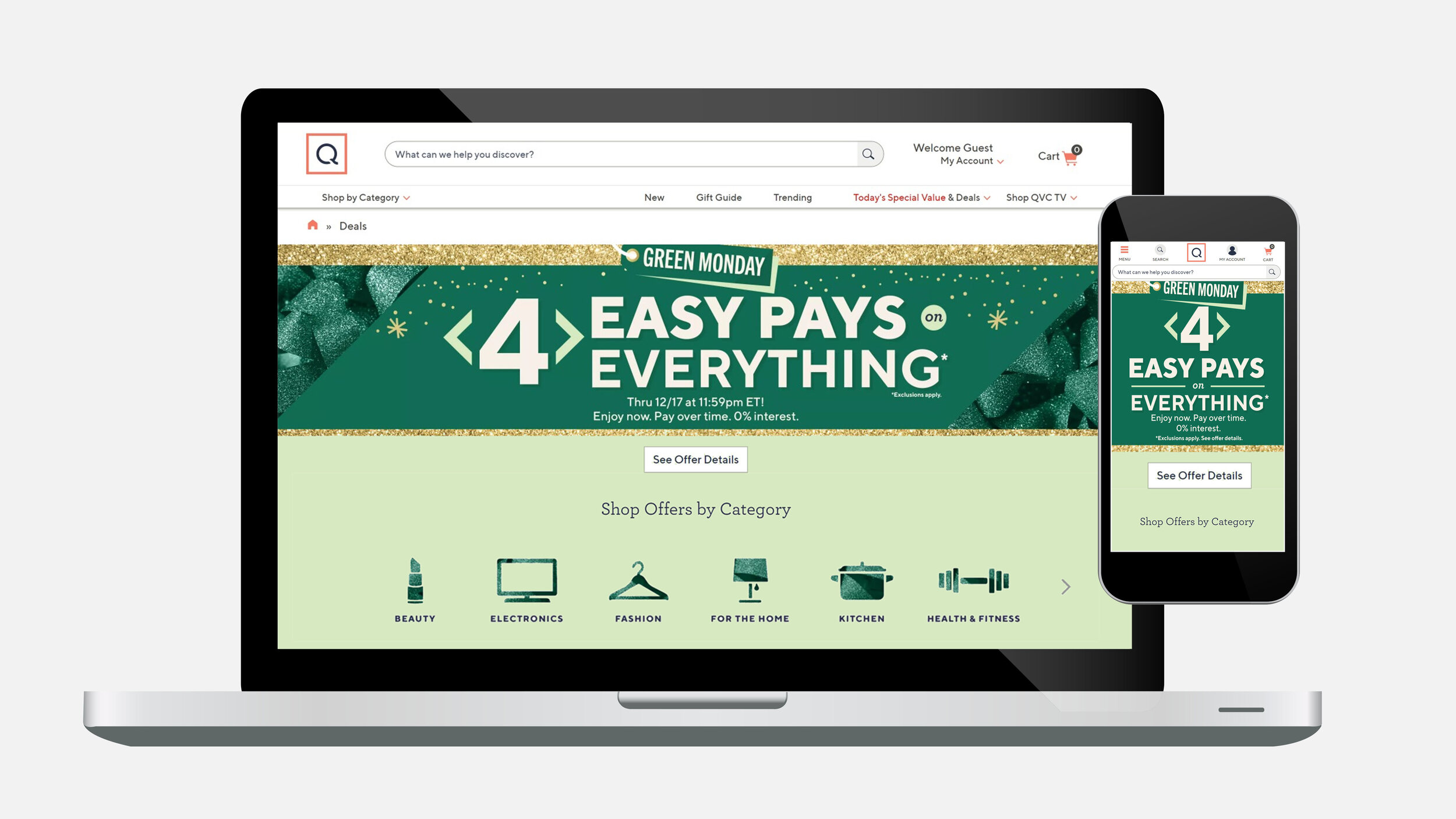In this detailed screenshot, the background is light gray, featuring images of a laptop and a cell phone. The laptop, encased in a sleek silver case with a distinct black outline, prominently displays a promotional banner on its screen. The banner in green and gold reads, "For Easy Pays Everything. Green Monday." The phrase "Green Monday" is styled to resemble a gift tag in green. Below this, there is additional text stating, "Through 12.17 at 11:59 p.m. Eastern Time. Enjoy Now. Pay Over Time. 0% interest." 

Further down on the screen, against a light green background, a white button labeled "See Offer Details" is visible. Below this section, there are different shopping categories, each represented by corresponding icons. Starting from the left, the categories include "Beauty" with an image of a lipstick, "Electronics" with an image of a laptop, "Fashion," "For the Home," "Kitchen," and "Health & Fitness." The layout is clear and structured, guiding the viewer through the various offers and options available.